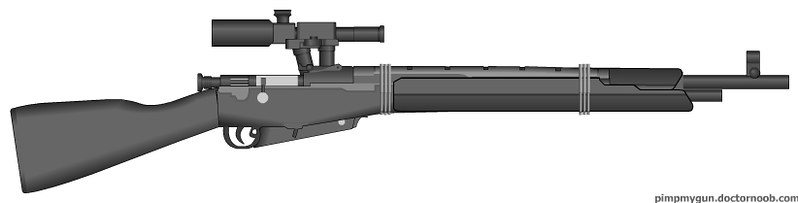This image features a detailed drawing of a black sniper rifle positioned horizontally against a completely white background, pointing towards the left. The rifle has a sleek, all-black design with a scope mounted on the top, also in black, which aligns perfectly with the end of the barrel. The stock is black, leading to the trigger and the long barrel, which has holes in it towards the muzzle. There are three gray bands around the rifle: one near the scope, another to the left of the middle, and one towards the muzzle. At the bottom right corner of the image, small dark gray text reads "pimpmygun.drnoob.com," showcasing the source of the drawing.